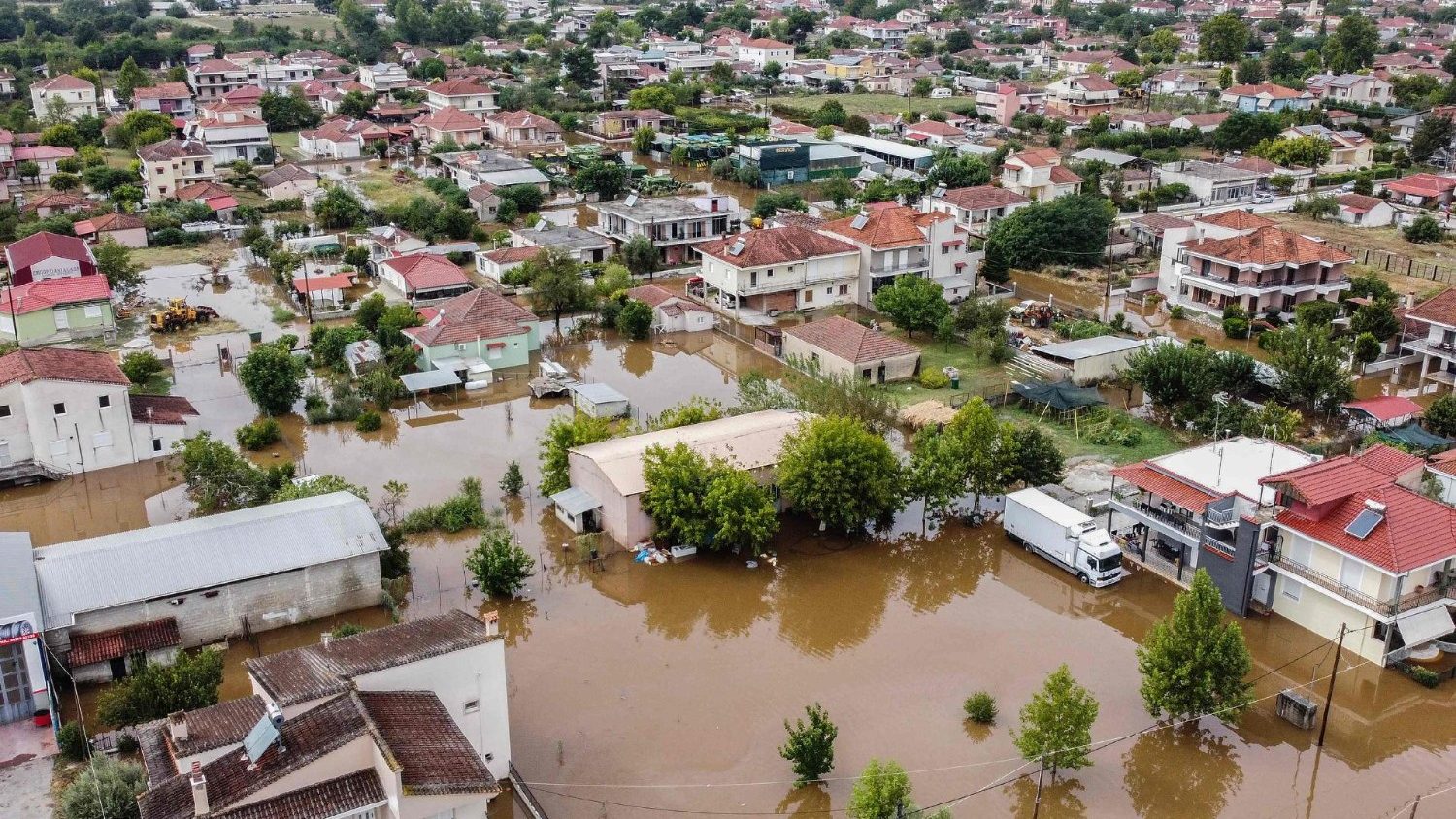An aerial view captures a large section of a town submerged under brown, stagnant floodwaters, likely from a heavy rain or hurricane. The image shows rooftops of various buildings, with a prominent number of them painted red. Interspersed among the structures are white and cream-colored houses, some with metal roofs of white, aluminum, or tan. The flooded area reveals several trees, power lines, and solar panels installed on some of the rooftops. The town’s layout includes both residential homes with distinct red roofs and possibly short condominiums or apartment buildings. A few large metal buildings can also be seen alongside a parked box truck partially submerged in the floodwaters. Overall, the devastation from the flooding is evident, affecting what looks like a substantial portion of this suburban area. There is no textual overlay in the image.